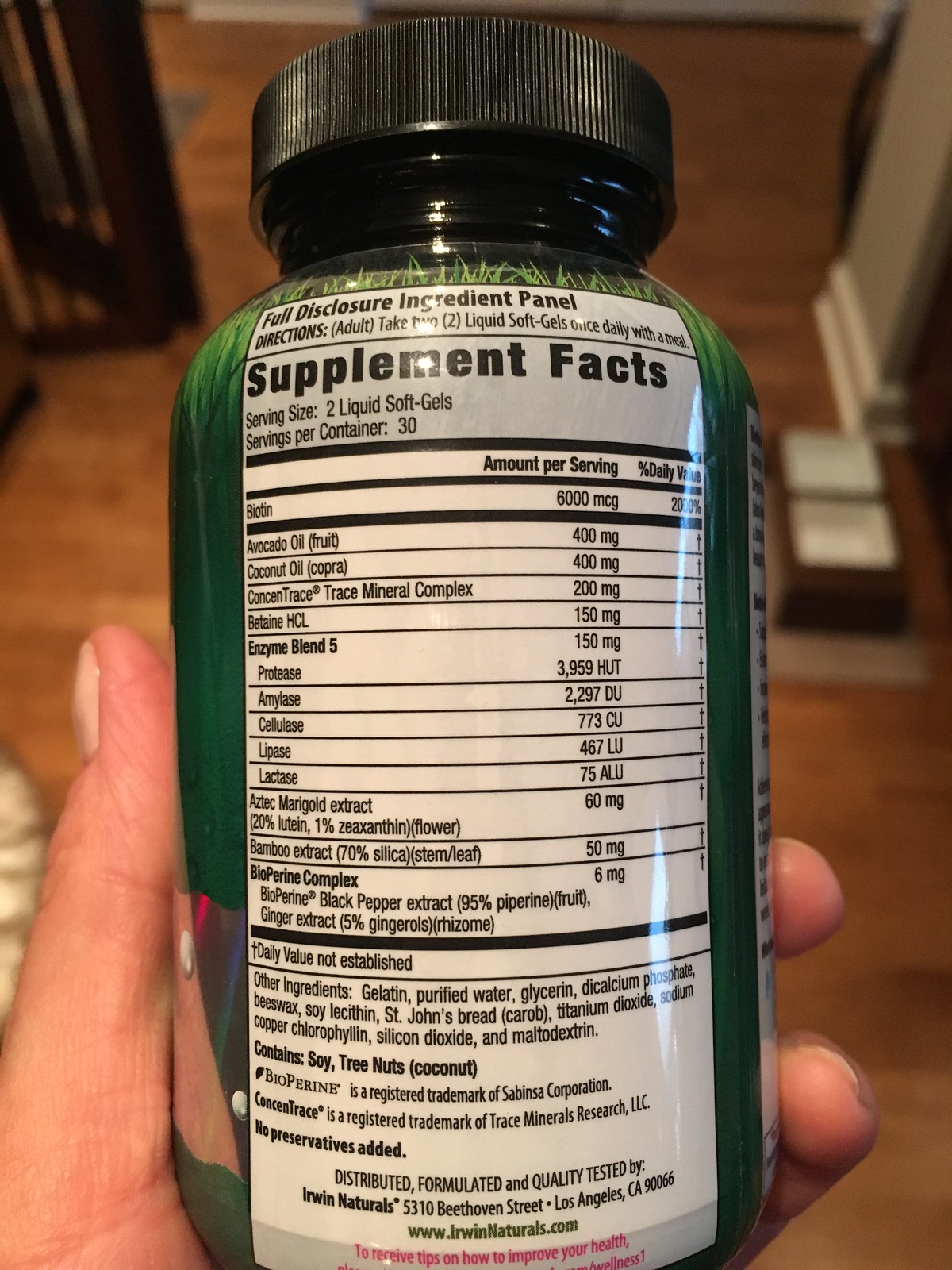In the image, a hand is prominently holding a green bottle with a white label and a black cap featuring ridges. The bottle has a white rectangular section on the label containing detailed supplement information. To the right of the hand, there are four wooden bowls arranged in a row. The background showcases a brown wall with a white wooden trim at the bottom, creating a contrasting yet harmonious look. The supplement facts on the bottle label include text indicating "Full Disclosure" at the top, and a variety of ingredients such as biotin, avocado oil, coconut oil, and numerous enzymes and extracts. The address for the distributor, Urban Naturals, is also listed along with their website. The overall aesthetic is rustic and sophisticated, blending natural elements with the detailed, informative presentation of the supplement bottle.